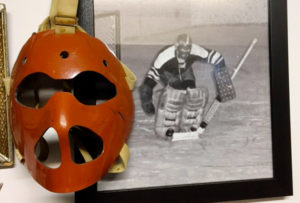In a small, rectangular image, a vintage black-and-white photograph is encased in a black frame. The photograph captures a hockey goalie in the midst of an action pose, bent over with a hockey stick in front of him, fully suited in leg pads and other gear. Draped over the left side of this framed picture is an old, rusty red face mask with eye holes and mouth holes, evoking the style of a traditional hockey mask. The overall scene suggests a poignant historical connection, possibly hinting that this mask once belonged to the goalie featured in the photograph.